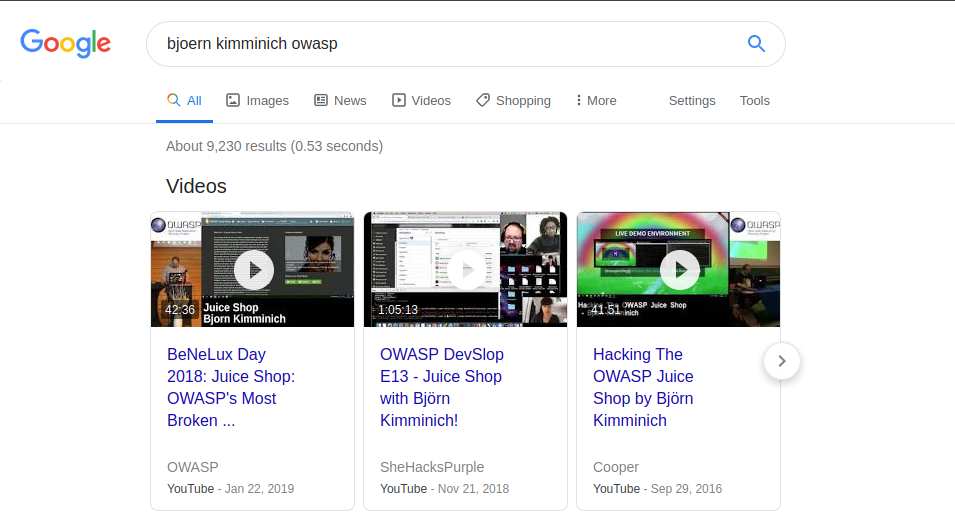The provided image is a Google search results page for "Bajoran Kimmich" and related keywords. At the top left, there's the multicolored Google logo, with the letters "G," "o," "o," "g," "l," and "e" in blue, red, yellow, blue, green, and red respectively. To the top right of the Google logo is the search bar icon, featuring a small magnifying glass. Below the search bar is the navigation menu, with "All" highlighted in blue, followed by options for "Images," "News," "Videos," "Shopping," "More," "Settings," and "Tools," all written in black text. The page reports receiving approximately 9,230 results in 0.53 seconds.

The main results section showcases three video thumbnails. The first thumbnail depicts a person standing at a podium with an orange backdrop. This video, titled "Juice Shop Bajoran Kimmich," includes a play button and the description "B-N-E-L-U-C-K-S-A-D-A-Y, 2018, Juice Shop," along with the source, YouTube, and the upload date, January 22, 2019.

The second thumbnail, labeled "OWASDEV D-V-S-L-O-P Episode 13: She Hacks," shows content from YouTube user SheHacksPurple, uploaded on November 21, 2018.

The third thumbnail is titled "Hacking the OWASP Juice Shop by Cooper," uploaded to YouTube on September 29, 2016.

To the right of these thumbnails is a right-arrow button, indicating that more similar video results can be viewed by navigating further.